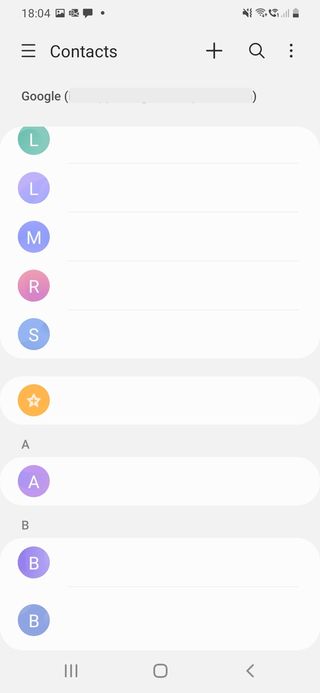The image is a detailed screenshot from someone's cell phone showing various elements of the device's interface. The entire background is light gray, with a darker gray strip at the top displaying the time, "18:04." Below this, there's a series of icons arranged horizontally:

1. A square icon featuring what appears to be a dark hill or mountain with a small dot at the top.
2. An envelope symbol.
3. An icon resembling a speech bubble or comment box.
4. A round circle icon.
5. A muted volume icon with a line through it.
6. A Wi-Fi signal icon.
7. A phone icon with signal waves emanating from it.
8. A cellular signal strength icon.
9. A battery icon.

Further down, there are three stacked horizontal lines with spaces in between, followed by the word "Contacts" in capital letters on the left, and to the right, there is a plus sign, a magnifying glass, and three vertical dots.

Below this, the word "Google" is displayed alongside a search bar enclosed in parentheses. The main white background features a series of colored circles, each containing a letter:

- A green circle with the letter "L."
- A light purple circle with the letter "L."
- A medium purple circle with the letter "M."
- A pink circle with the letter "R."
- A blue-purple circle with the letter "S."

After a small space, there's a yellow circle with a star symbol. Below this, other circles contain additional letters:

- An "A" within a white circle bordered by purple.
- A "B" within a purple circle inside the white background.
- Another "B" within a blue-purple circle.

Each circle and letter combination stands out, positioned against the white background, to clearly differentiate each contact.